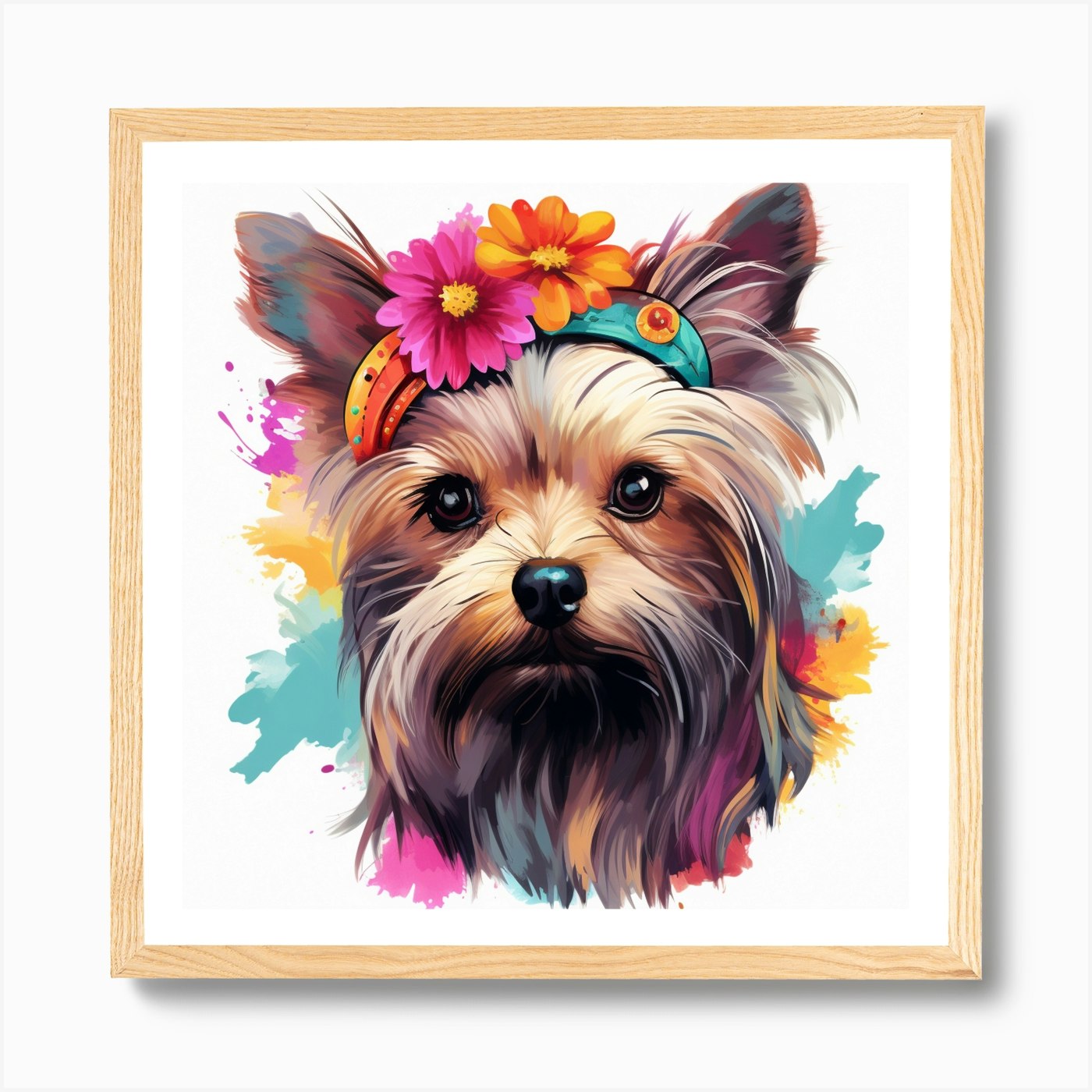This digital artwork captures a close-up of a small Yorkie dog adorned with a vibrant, bohemian-style headband. The dog's soft coat blends shades of blonde, light brown, and tan with strikingly large, dark brown eyes and detailed features, including long eyebrows, ear tufts, and a distinguished beard. Its headband, primarily turquoise and orange, is embellished with two daisy-like flowers—one bright pink with a yellow center and the other orange with a yellow center. The background features splashes of watercolor in bright pink, yellow, and blue, creating an artistic halo around the dog against a stark white backdrop. The image is framed in a pale, light oak wood, emphasizing the colorful and playful nature of the scene.